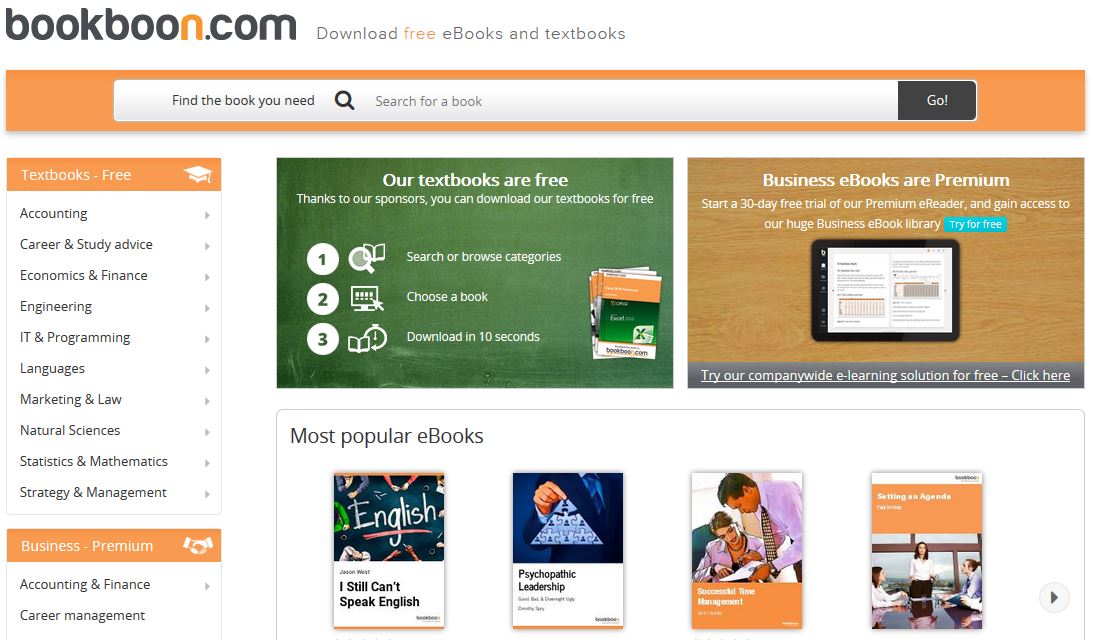The image is from Bookboon.com, featuring their logo prominently at the top. The website name "Bookboon" is displayed in a large, bold black font, with the "N" in "boon" highlighted in a yellowish-orange color. Following the logo, ".com" is also in bold and lowercase. Below the logo, the text "Download Free eBooks and Textbooks" is shown, with "Free" in the same yellowish-orange color.

An orange banner located beneath the introductory text contains a search bar with a magnifying glass icon and the prompt "Find the book you need." Adjacent to the search bar is a dark gray button that says "Go!" in bold.

On the left side of the image, a vertical column features a series of banners and categories. The first banner reads "Textbooks Free" and includes a graphic of a mortarboard hat with a tassel. The categories listed under this section include Accounting, Career, Economics, Engineering, IT, Languages, Marketing & Law, Natural Sciences, Statistics & Mathematics, and Strategy & Management.

Another banner below this section states "Business Premium" accompanied by an image of a handshake. The brief, partially obscured categories under this heading include Accounting and Finance, and Career Management.

In the middle of the image, there are two sections with the captions "Our Textbooks are Free" and "Business eBooks are Premium." Underneath, the headline "Most Popular eBooks" introduces four highlighted books: "I Still Can’t Speak English," "Psychopathic Leadership," an unreadable title, and "Setting an Agenda."